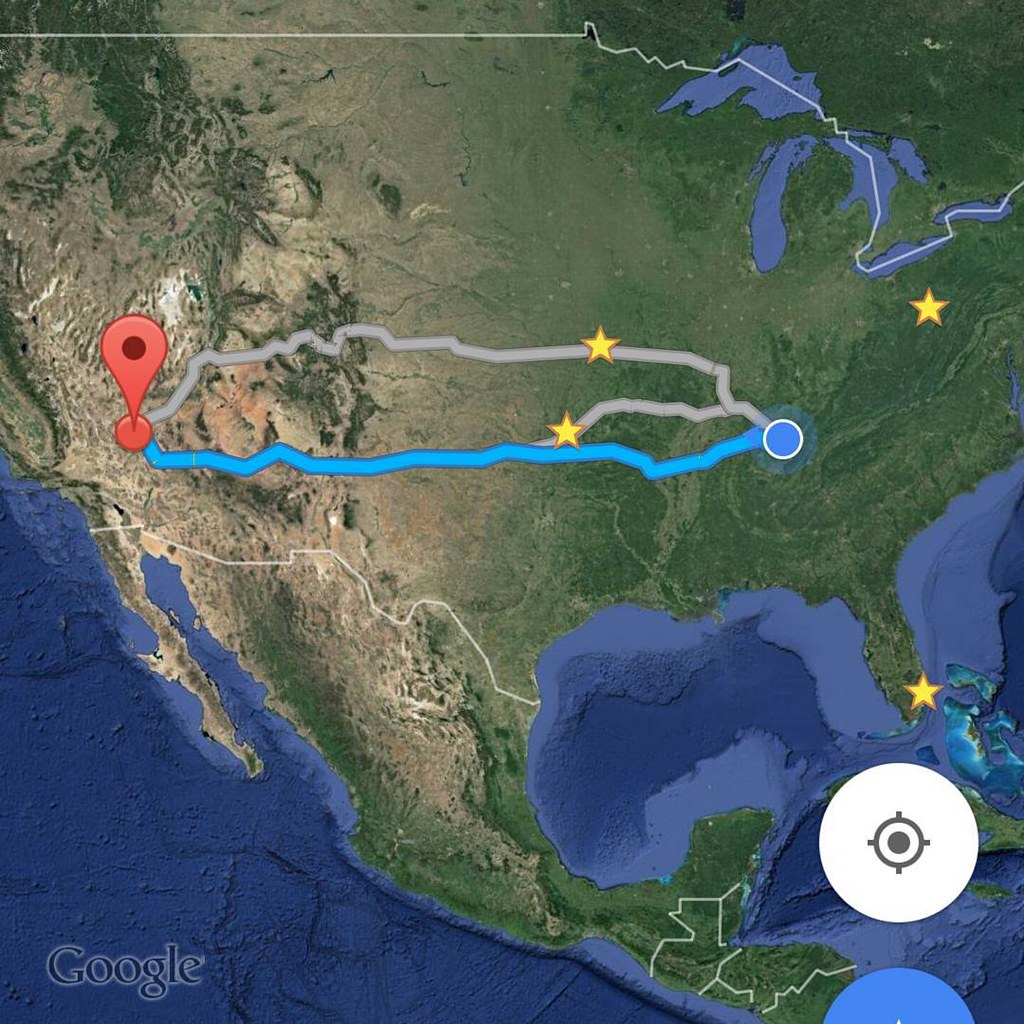The square image appears to be a screenshot from Google Maps, showcasing a detailed route plan from the eastern region, likely Tennessee, to Las Vegas. The map covers a broad satellite view of North America, depicting the United States, parts of Mexico, and Central America. The main route is highlighted in blue, indicating the fastest path, while alternate longer routes are shown in gray. The map also features distinct outlines of countries and regions in white and highlights key water bodies like the Great Lakes and the Pacific, Gulf of Mexico, and Atlantic Oceans. Additional elements include yellow stars marking locations in Florida and two places in the Midwest, possibly Ohio or New York State. The destination is marked with a red pin, and the route originates from a blue circle, denoting the starting point.